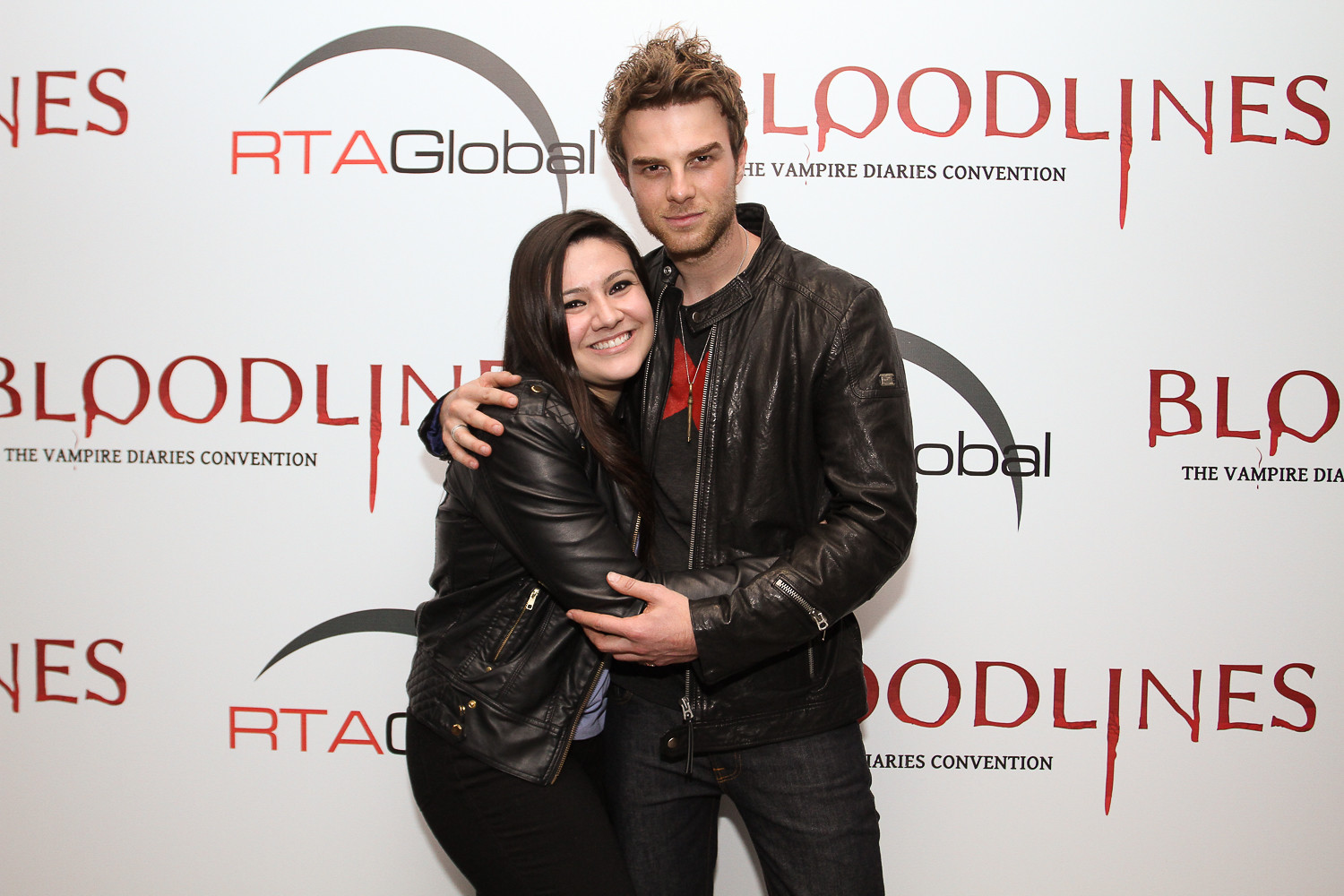In the center of the image, a young woman and a young man pose in front of a large poster backdrop adorned with various texts and designs. The backdrop prominently features the title "Bloodlines" in blood-red lettering, with repeated appearances of "RTA Global" in black and red, and references to "The Vampire Diaries Convention" further enhancing the thematic setting. 

Both individuals are dressed in black leather jackets, exuding a sleek and coordinated look. The woman, positioned slightly hunched as she embraces the man around his waist, beams directly at the viewer. She is sporting long, below-the-shoulder brown hair, a black blouse underneath her jacket, and black pants. Her posture conveys warmth and affection as she rests her head against the man's chest.

The man, with wavy, now spiked blonde hair, reciprocates by draping his right arm around her shoulders and gently holding her left elbow with his left hand. He is dressed in a black t-shirt that features a red insignia across the chest and pairs it with dark blue jeans. His subtle smile adds to the intimate atmosphere of the photo. 

Adding to the scene's richness, a boomerang-like graphic appears above the repeated text, and subtle smears and key details contribute to the overall authenticity and emotion captured in this promotional yet intimate moment.